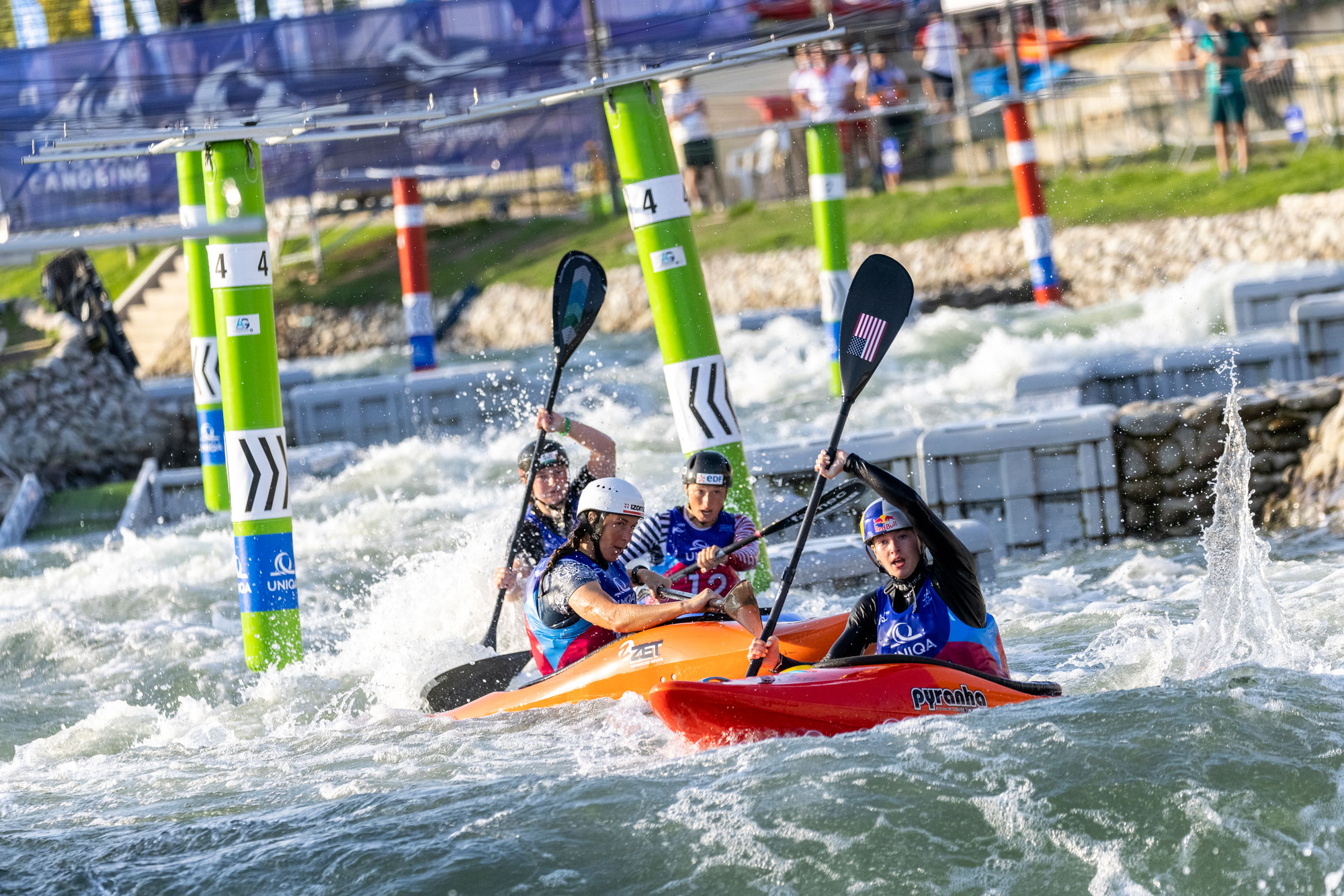The image captures a dynamic whitewater kayaking race on what appears to be a man-made course. Four kayakers navigate the light green rapids, creating substantial white splashes. In the foreground, a girl in an orange kayak labeled "PYRANHA" with black letters holds a black paddle adorned with an American flag sticker aloft. She wears a blue suit and black sleeves. Close behind her, another girl in an orange kayak with the label "ZET" in black wields her paddle, donning a light blue uniform with dark blue sleeves and a white helmet. Further back to the left, a girl with a black helmet and blue-and-white striped sleeves heads straight towards the camera. In the very rear, another kayaker in a black-topped canoe raises their paddle high, wearing a black helmet and shirt. Green poles with white labels and the number four mark the course, and additional red poles with similar markings are also present. These racers are cheered on by spectators lining the grassy, stone-formed shoreline, highlighting the competitive and organized nature of this thrilling kayaking event.